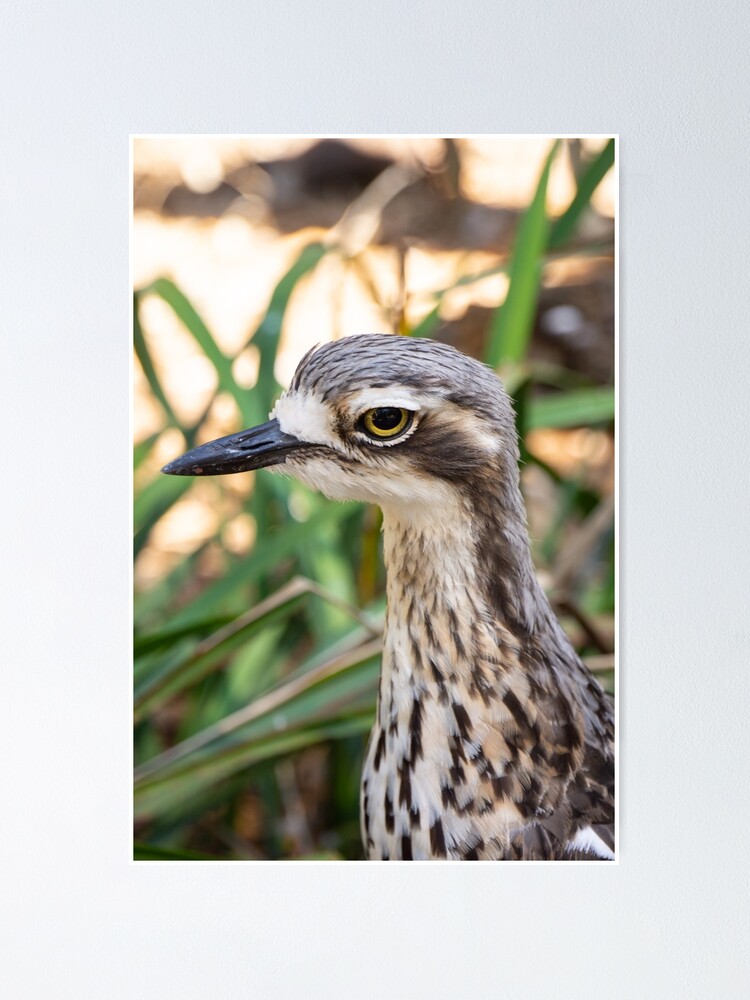This close-up image captures a detailed profile of a bird's head and neck, focusing on its distinctive features. The bird, with a noticeably long, slender neck, boasts a medium-sized, sharp black beak that is reminiscent of a spear point. Its eye, black with a striking yellow ring, is set against a white surrounding area. The head and upper body display a mix of grey and white feathers adorned with small black spots and streaks, especially noticeable on the chest. The bird's upper back feathers appear darker, while the lower front, around the chin and nose, remains predominantly white. The feather pattern also includes some brown elements. The blurred background features elongated green leaves and vines, indicating an outdoor, sunlit environment. The foliage and bright, unfocused backdrop suggest the bird's natural habitat in a grassy, sunlit area.